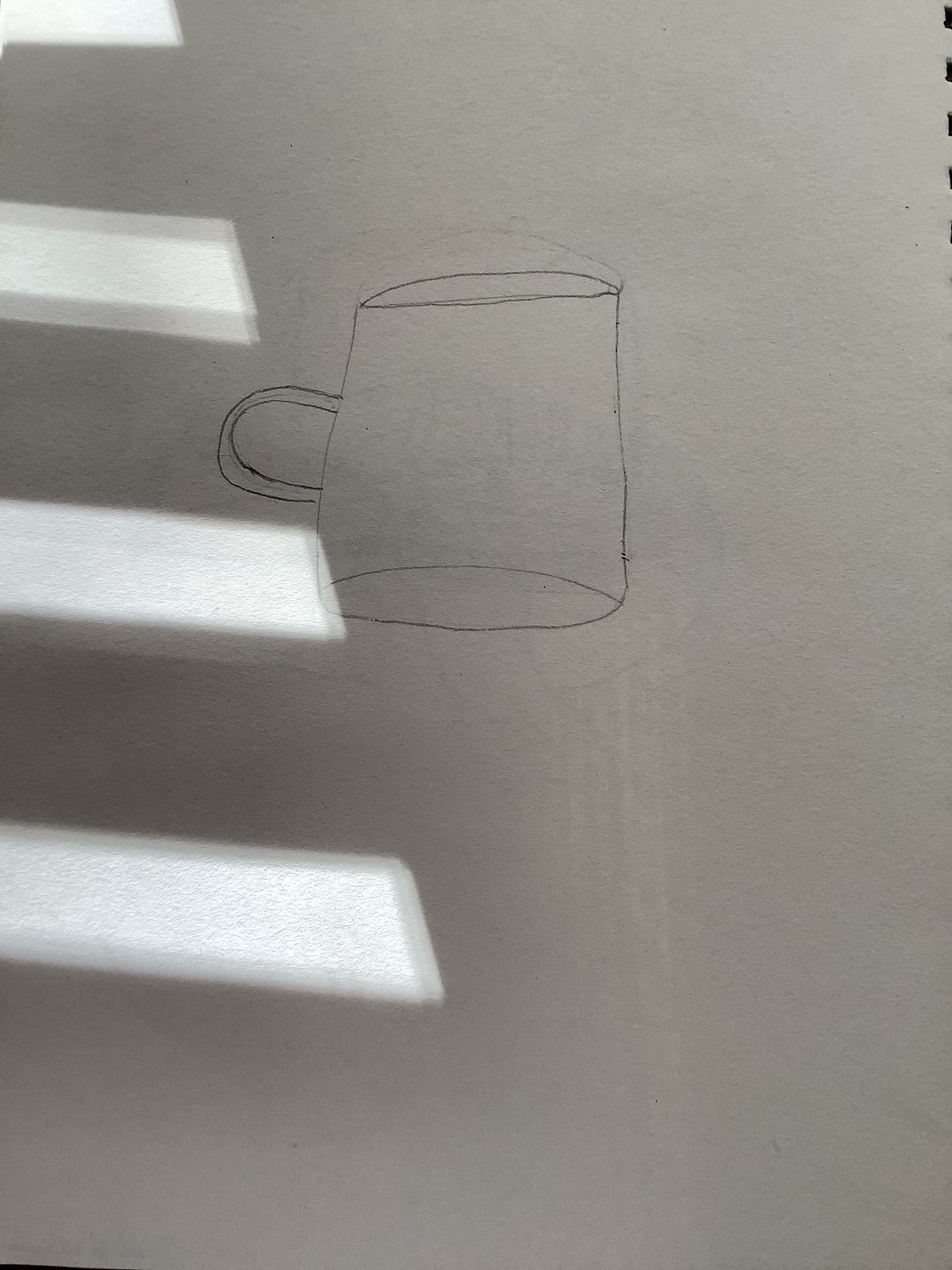This image showcases a pencil drawing on gray, unlined paper, which is part of a spiral-bound sketchbook, as indicated by the visible spirals in the upper right corner. Light from nearby blinds creates four distinct lines across the left side of the paper, suggesting sunlight filtering through. The artwork itself features a simple sketch of a mug or cup, rendered to appear three-dimensional with a circular base and top, connected by two vertical lines. A small double 'C' on the right side forms the handle. The drawing is in pencil, without any added color or shading, capturing a clear and minimalist design.